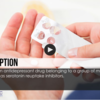The image depicts a display screen featuring a tutorial video for a website. At the bottom of the image, part of a wrist is visible against a blue background on the right. Above this section, there is a black rectangular area with very blurry white text inside it. The middle portion of the image showcases a white background extending from side to side, with the letters "P-T-I-O-N" in black on the left side. Centrally positioned above this, there is a black circle containing a play button. The background displays the underside of a hand on the left, and another hand gripping a remote control with a thumb and index finger on the right. The remote control has four buttons on its top. The rest of the background is light gray, with a hint of faded yellow towards the top.